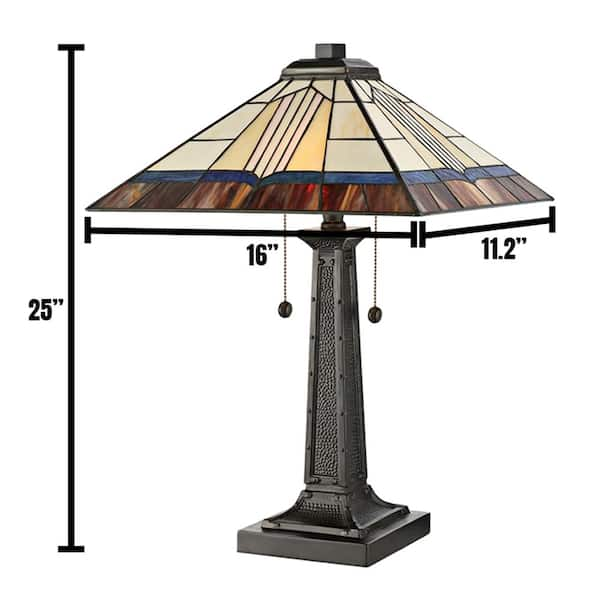This image depicts a detailed view of a lovely table lamp against a solid white background. The lamp features a sturdy, dark gray metal base with a square bottom, narrow stem, and a taller arm decorated with a bumpy, circular texture and perforations along the trim. The total height of the lamp is indicated to be 25 inches, marked by a vertical black line with tiny horizontal lines at each end for precision.

The lamp boasts a beautiful stained glass lampshade that is distinctly geometric with sections of various colors and shapes, including triangles, squares, and trapezoids. The shade is four-sided, tapering to a square point at the top, which is capped with a dark gray stem. The base of the shade is primarily a rich chocolatey brown with brown lines, bordered by a blue trim, followed by segments of tan, bone white, and hints of blue above. Measuring 16 inches across the front and 11.2 inches across the side, this exquisite stained glass lampshade adds an artistic and colorful touch to the otherwise metallic and structured lamp.